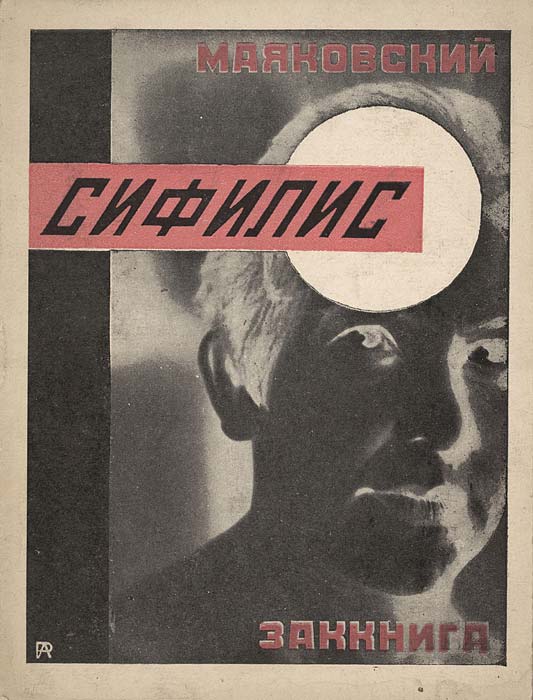The image appears to be a Russian magazine cover or possibly a book or movie poster featuring Cyrillic text. At the top of the page, there are several words in Russian, starting with characters resembling "M A," followed by a backward "R" or "K," "O B C K," and two backward "N"s. A faded red banner stretches across the middle of the page, overlaying the forehead of a person in the image. The banner contains Cyrillic characters, including a "C" and a backward "N," among others. The central figure is a man with medium-length hair, depicted in a heavily stylized, black-and-white, high-contrast photograph that makes him look almost like a negative image. His eyes and mouth are strikingly illuminated, creating an eerie effect as if they are popping out towards the viewer. The background of the image is in shades of black, white, and gray, enhancing the dramatic contrast. At the bottom, more Cyrillic text is visible but difficult to decipher, ending in characters that include numbers and potentially an upside-down "L." On the man's forehead, below the red banner, there is a circular mark, either red or white. The overall composition gives the cover a mysterious and intense visual impact.